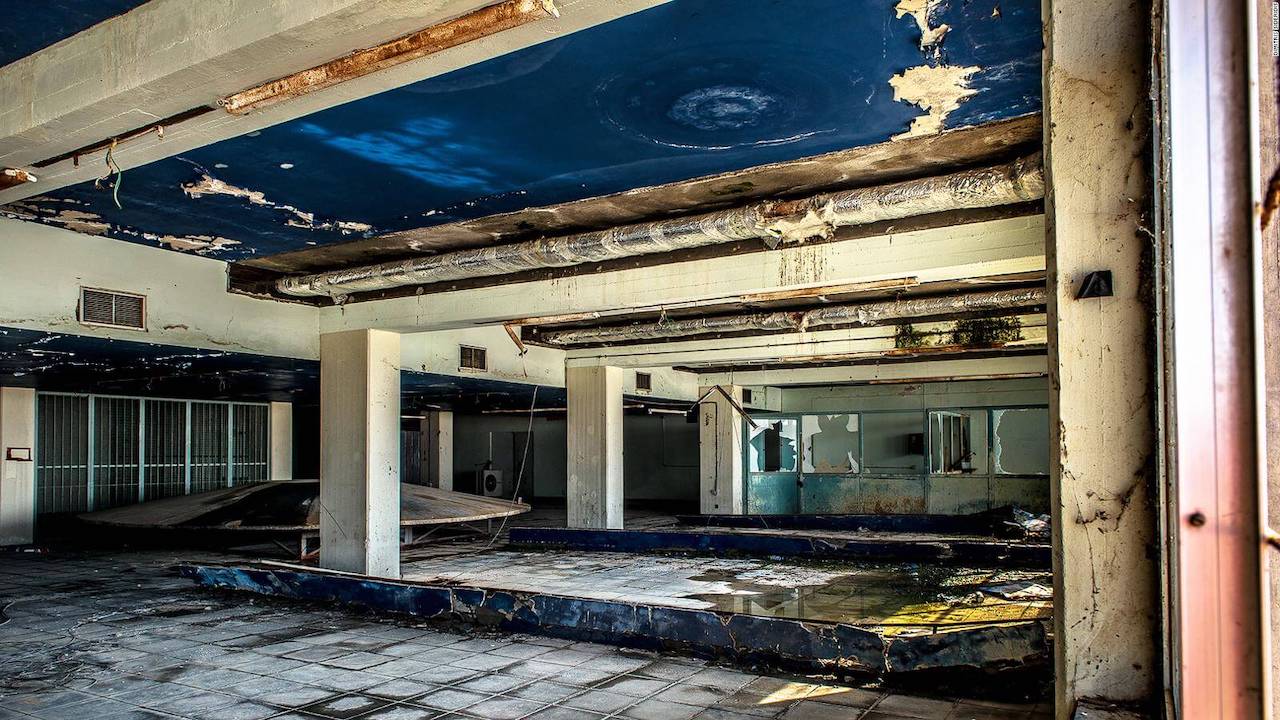The photograph depicts the deteriorated interior of a severely abandoned building, reminiscent of a parking structure. The scene reveals several square concrete pillars and beams that remain standing amid the decay. The entire space is in a severe state of disrepair, with visible damage including broken and shattered windows, missing paint and plaster, and notably, parts of the ceiling are caving in. There is an observable array of exposed HVAC ducts, while numerous sections are rotting or severely weathered.

To the right, a distance away, there appears to be a small office space potentially used by attendants or other workers in the past. The left side shows bars, resembling those of a jail cell, which could lead to another area or the exterior. The floor is a dirty, torn-up tile surface, marred with wet spots and grime, indicating long-term neglect and lack of human presence. Natural daylight seeps in through the remaining panes of glass, emphasizing the contrast between the sunlit exterior and the dim, desolate interior.